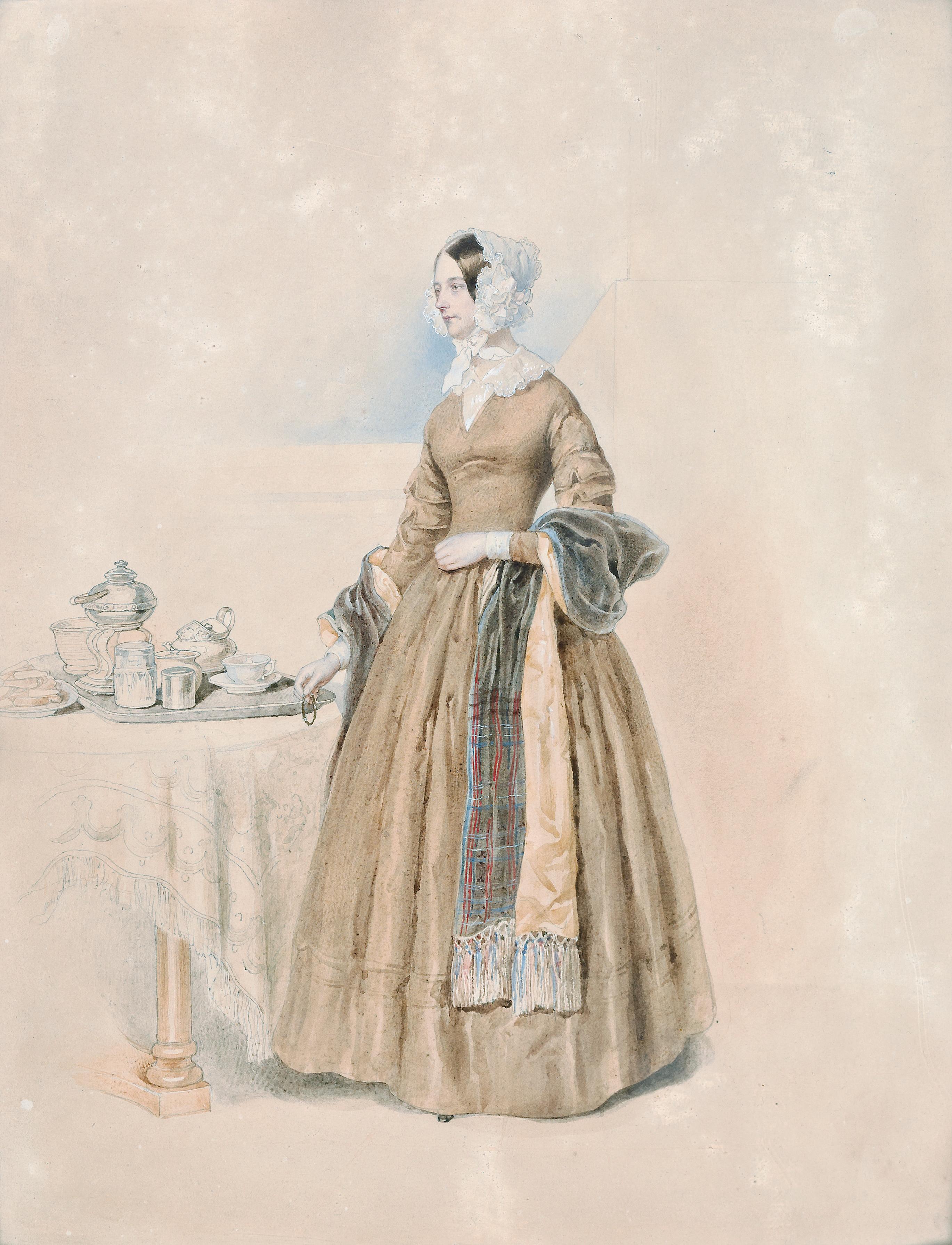This detailed watercolor and pencil painting depicts a woman of apparent nobility from a past century, dressed in elegant, upper-class attire. She wears a long, floor-length beige dress with white ruffles around her neck, exuding sophistication. Her head is adorned with a white, frilly headdress that ties neatly under her chin, complementing the white gloves she wears. Draped gracefully over her arms is a plaid gray and red shawl with a white edge, which also wraps around her waist. The scene is set against a beige-toned background with subtle hints of baby blue. To her left stands a round table with a prominent yellow leg, draped in a white and blue lace tablecloth. This table is intricately arranged with various tea-related items, including teapots, cups, glasses, and a tray, along with a plate of bread, creating a refined tea-time setting. The entirety of the painting maintains a delicate beige and white theme, emphasizing the period elegance.